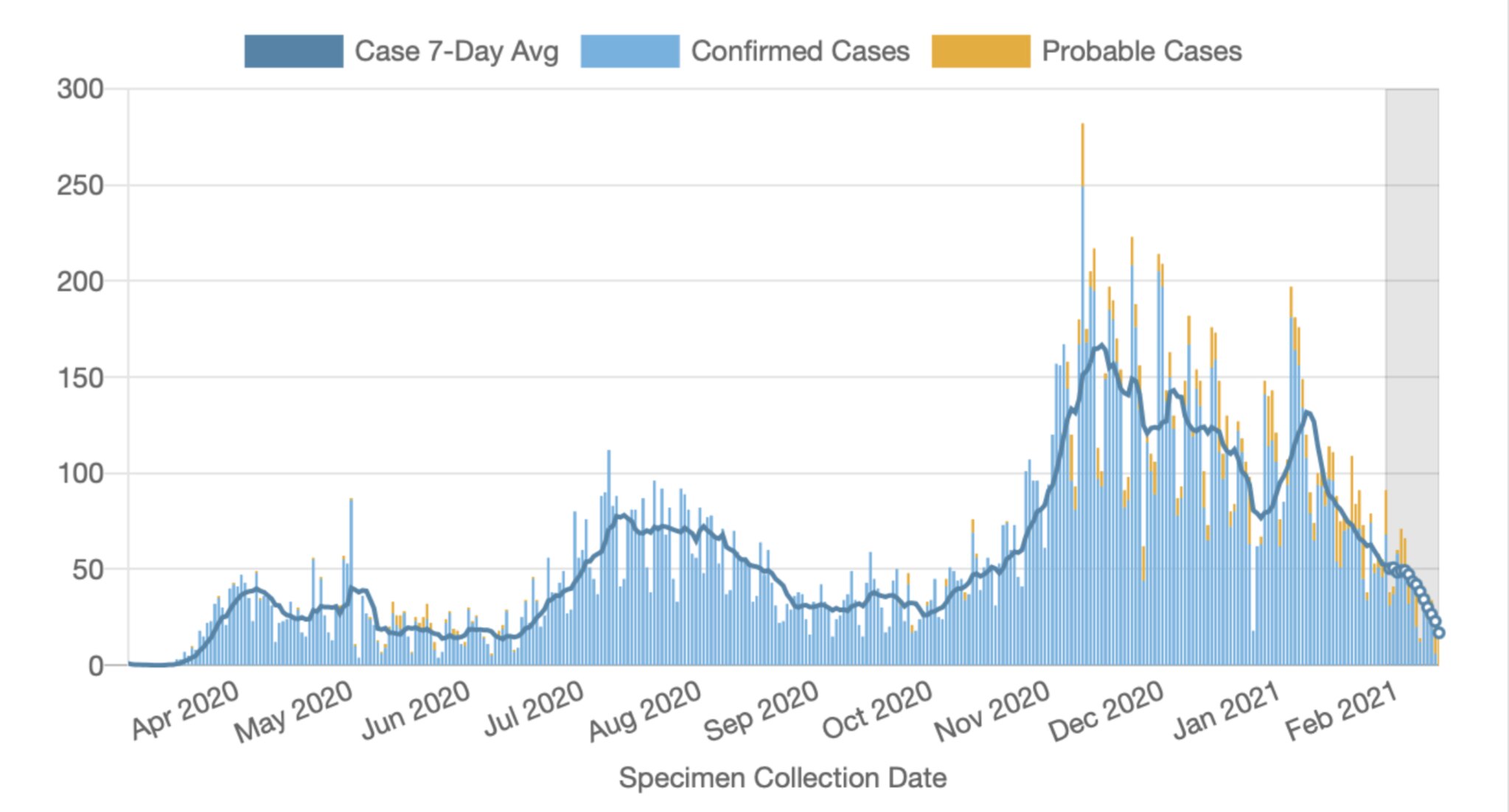This horizontally aligned rectangular line graph displays the trend of specimen collection data over time. The x-axis represents specimen collection dates, ranging from April 2020 to February 2021, with ticks each month. The y-axis shows the number of specimens collected, ranging from 0 to 300 in increments of 50.

The graph includes three color-coded elements: a dark blue line indicating the 7-day average of cases, a medium blue area representing confirmed cases, and an orange area for probable cases. The dark blue line starts low, follows a series of hills and valleys, peaks to around 275, then dips before slightly increasing and finally declining again.

The confirmed cases are illustrated with numerous vertical spikes that follow a similar overall trend to the 7-day average line. The probable cases, shaded orange, prominently appear towards the end, overlapping with the tips of the confirmed case spikes. This visual representation provides a detailed view of the fluctuating trends in specimen collections over the specified period.